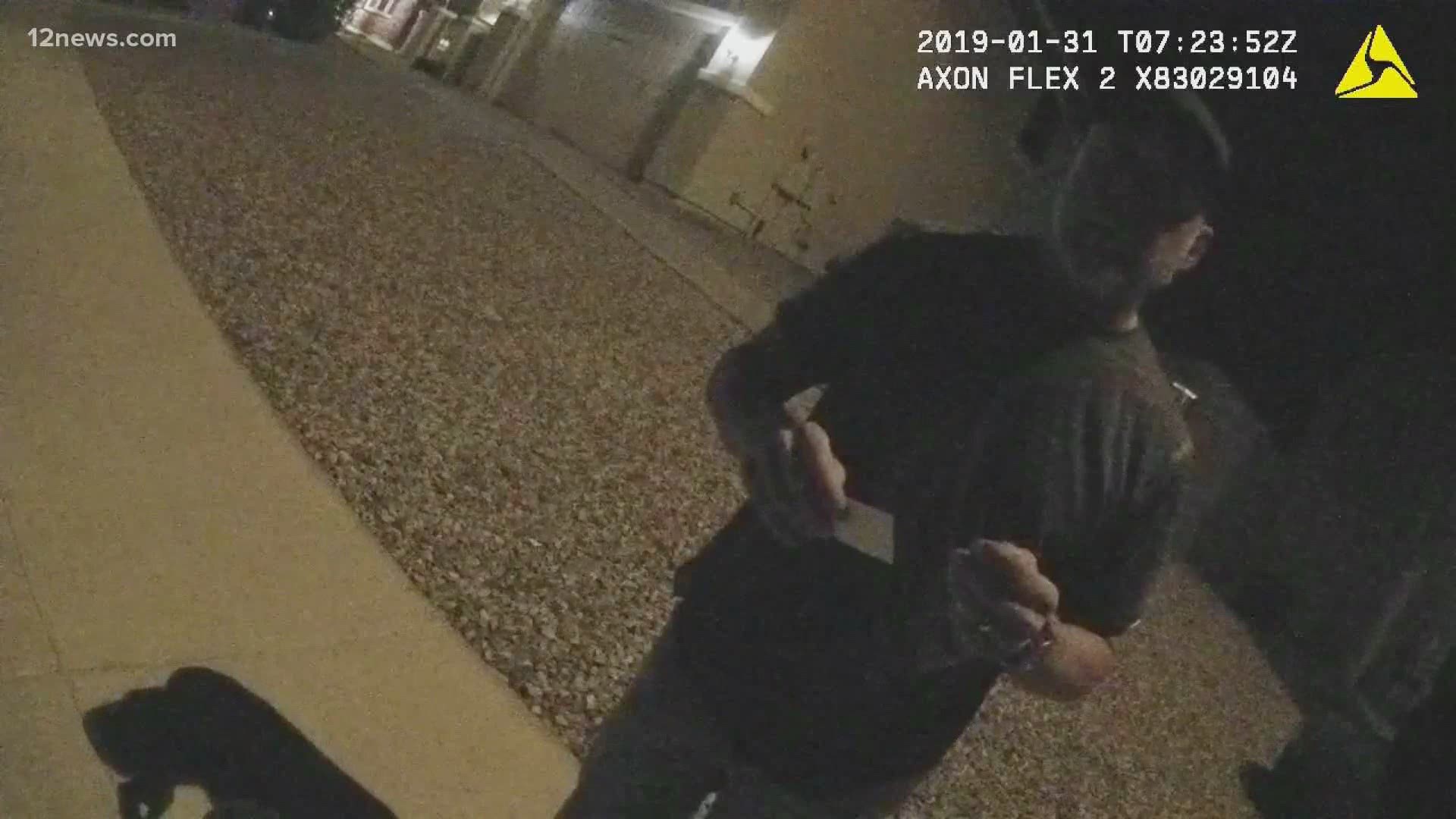This image appears to be captured from a body camera, identifiable by the "AXON Flex 2" watermark on the upper right. In the upper left corner, there is an "12news.com" watermark. The timestamp "2019-01-31 T07:23:52Z" is displayed at the top right. The right side of the image features a man wearing a black hat and a black short-sleeved t-shirt. He holds a piece of paper in his right hand and is wearing a watch on his left wrist. He is looking directly at the camera. The setting includes a large garage door, a grassy area, and a sidewalk. The background suggests the exterior of a building, and a distinct yellow triangular-shaped object can be seen to the right of the frame. A pronounced shadow is visible on the ground to the left of the man.